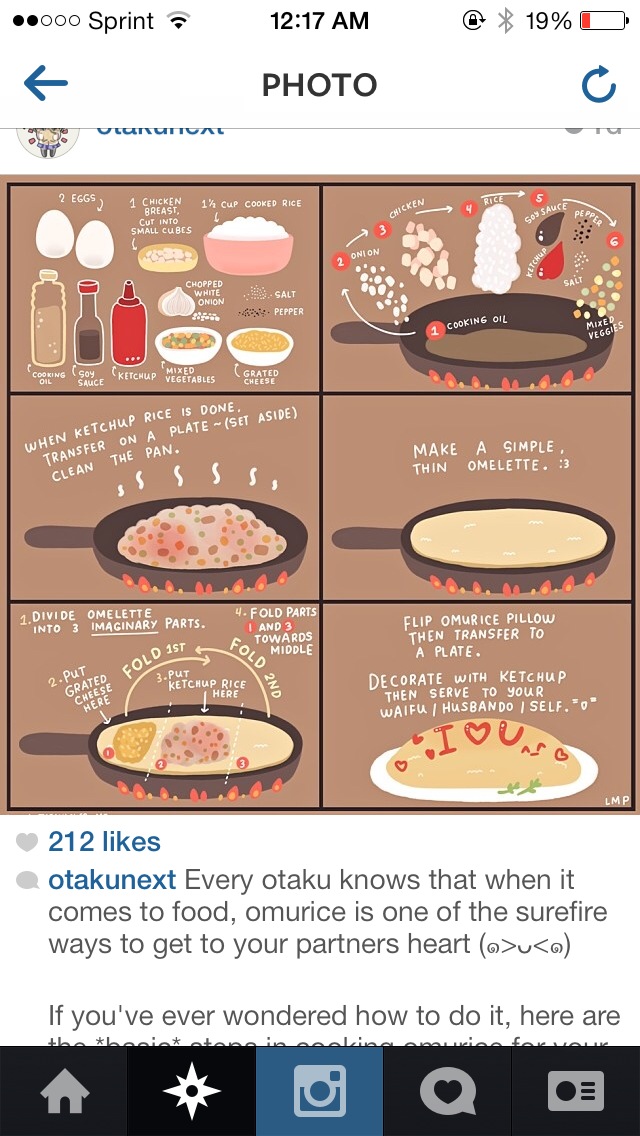This image is a detailed, step-by-step animated recipe screenshot for making Omurice, captured from a smartphone with Sprint service at 12:17 AM, showing a 19% battery level. The Instagram post by Otaku Next, which has garnered 222 likes, illustrates the process across six frames:

1. The top left frame displays the necessary ingredients: two eggs, cubed chicken breasts, cooked rice, cooking oil, soy sauce, ketchup, and mixed vegetables.
2. The top right frame shows the ingredients being combined in a pan with cooking oil.
3. The middle left frame instructs to transfer the cooked rice mixed with ketchup to a plate and set aside.
4. The middle right frame advises making a thin omelet.
5. The bottom left frame depicts dividing and folding the omelet into three sections.
6. The bottom right frame reveals the final product: an omelet beautifully decorated with ketchup, spelling out "I ♥ you."

This recipe is celebrated as a beloved dish among otakus, described in the post as a surefire way to win your partner's heart.